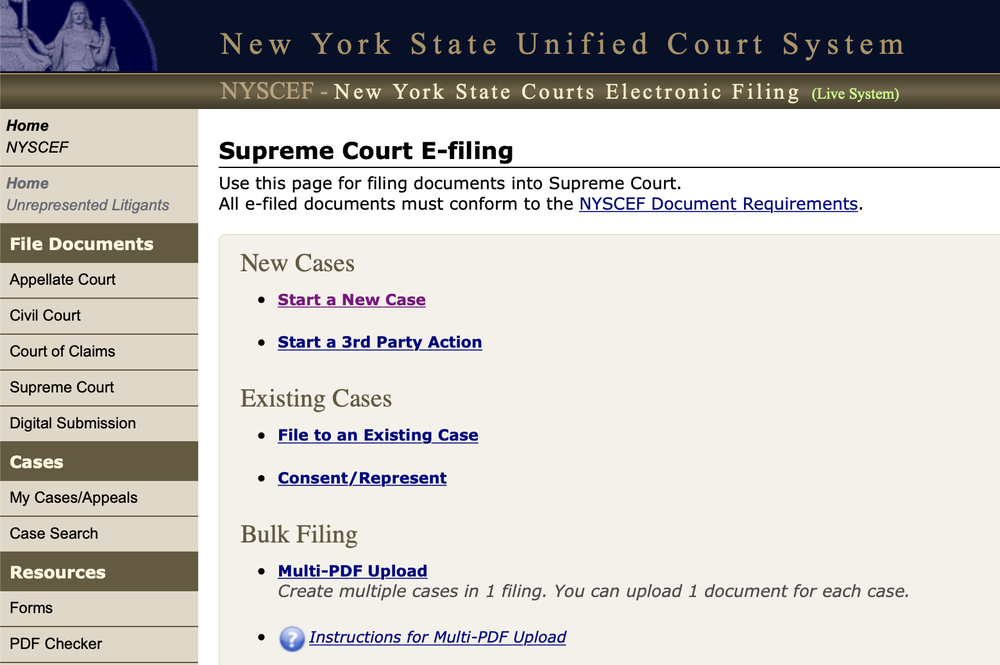This image captures a webpage from the New York State Unified Court System's electronic filing platform, known as NYSCEF, specifically its live system interface. On the left side of the screen, there is a menu with several sections. The first section includes the "Home" option and a category for "Unrepresented Litigants." Below this, in the "File Documents" section, there are five subcategories: Appellate Court, Civil Court, Court of Claims, Supreme Court, and Digital Submission.

Moving down, the "Cases" section offers "My Cases/Appeals" and "Case Search" options. The final section, "Resources," includes "Forms" and a "PDF Checker."

In the center of the screen, a prominent header reads "Supreme Court E-Filing." Beneath it is a directive for users: "Use this page for filing documents into Supreme Court. All e-filed documents must conform to the NYSCEF document requirements." This text is underlined and displayed in a bluish-purple color, indicating it is a clickable link.

Directly below, the "New Cases" section features two bullet points: "Start a New Case" and "Start a Third-Party Action." Additionally, options for managing "Existing Cases" and initiating "Bulk Filing" are also visible.